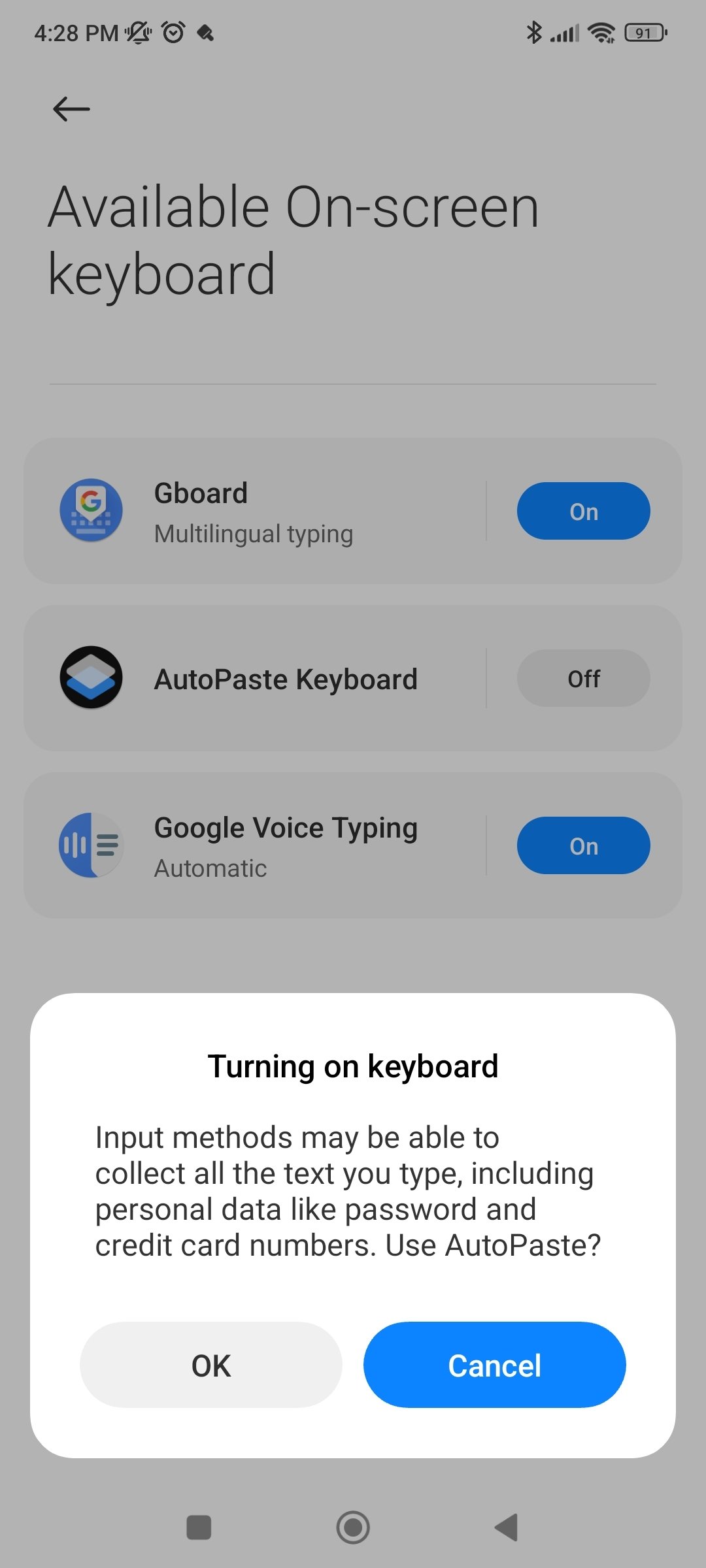The image is a screenshot taken from a smartphone, showcasing a configuration screen for available input methods. The background color of the screen is gray. 

At the top left corner, the time displays as 4:28 PM. On the top right, various status icons are visible: a battery icon indicating a 91% charge, a Wi-Fi signal logo, a wireless connection icon, and a Bluetooth icon.

Below the status bar, the heading "Available on Screen Keyboard" is written in a gray font. Three options are listed beneath this heading:

1. **G-Board:** Indicated to the right with a blue oval button that reads "On" in white text.
2. **Auto-Paste Keyboard:** Accompanied by a gray oval button displaying "Off" in dark gray text.
3. **Google Voice Typing:** Also featuring a blue oval button that says "On" in white text.

Toward the bottom of the screen, there is a white rectangle with rounded corners, containing explanatory text regarding the "Turning On Keyboard." Within this rectangle, in the lower-left corner, a gray button labeled "OK" is visible. On the lower-right corner, there is a blue oblong button with the word "Cancel" written in white.